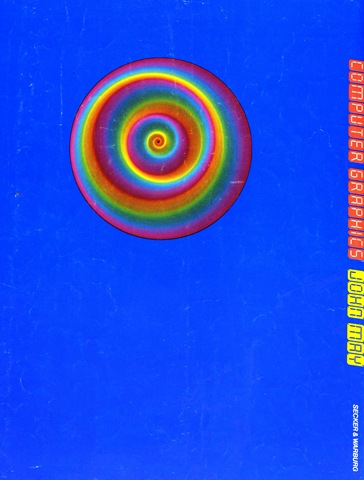The image is a vertical digital composition featuring a prominent circle in the middle, containing a vibrant, rainbow-colored spiral that transitions through hues of yellow, purple, blue, orange, red, and various shades in between. The spiral pattern intricately winds towards the center, creating a captivating focal point against the royal blue background, which appears slightly scratched and faded in areas. Along the right edge, vertically aligned text reads "Computer Graphics," with each letter set in orange uppercase over separate rectangles. Adjacent to this, another set of yellow rectangles houses blue uppercase letters, spelling out "John May." Beneath these, in smaller white text, "Secker and Warburg" is also oriented vertically towards the bottom right corner. This combination of vivid colors and structured text creates a visually striking and detailed graphic.